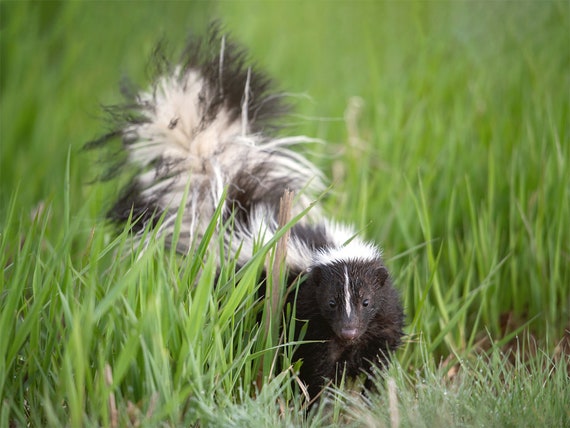In this professional outdoor photograph, a skunk takes center stage as it walks through a lush, tall field of grass. The vibrant green grass, interspersed with white tips and morning dew droplets, adds a dynamic texture to the foreground, creating a striking contrast against the blurred background hues of greens, yellows, and beiges. The skunk itself is captured in exquisite detail: its small, black eyes gaze directly at the camera, framed by a distinctive white stripe running from the tip of its nose up to its forehead and between its ears. The skunk's body is marked by two prominent white stripes down its back, while its plump, fluffy tail— mostly white with patches of black fur—stands upright in a charmingly disheveled manner. The skunk’s natural beauty and the serenity of its weedy, natural surroundings paint a compelling and endearing portrait of wildlife in its habitat.